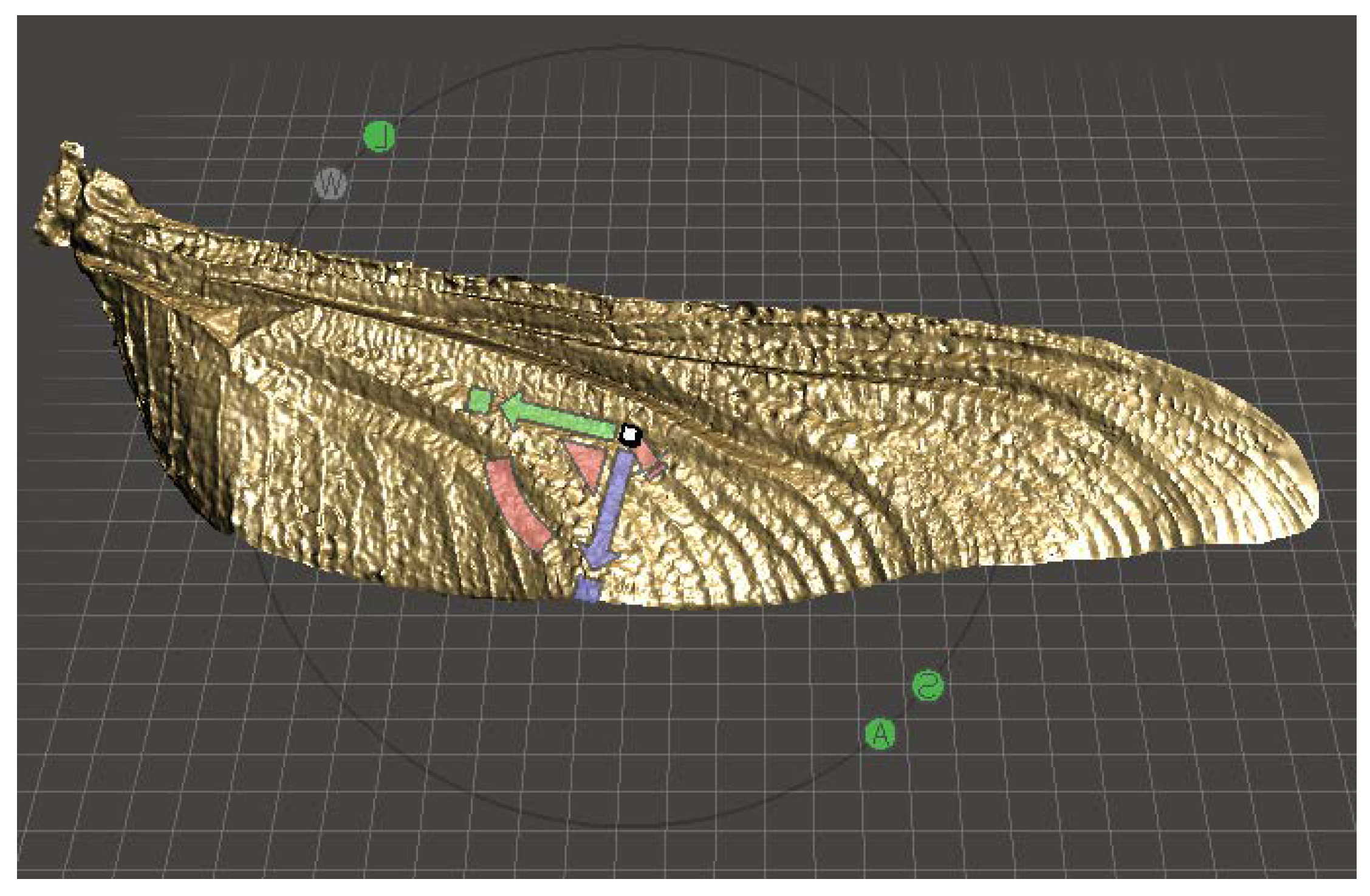The image is a horizontal, rectangular photograph featuring an intricate, gold-colored object that resembles a leaf or possibly an insect wing. The object has a curving, elongated shape with vein-like ribs, making it look like it could function as a handle. It rests on a back surface adorned with a white grid pattern of horizontal and vertical lines, creating a checkerboard effect. Surrounding the gold object, there are additional design elements, including dark and lighter brown lines extending from the base and forming a complex, segmented structure towards the end. Notably, there are two small green dots on the gold object, adding to the detailed craftsmanship. The image also includes UI interface elements: a dark gray circle with various letters around it, and some lines equipped with arrows, suggesting the photograph might be a 3D model within a digital application.